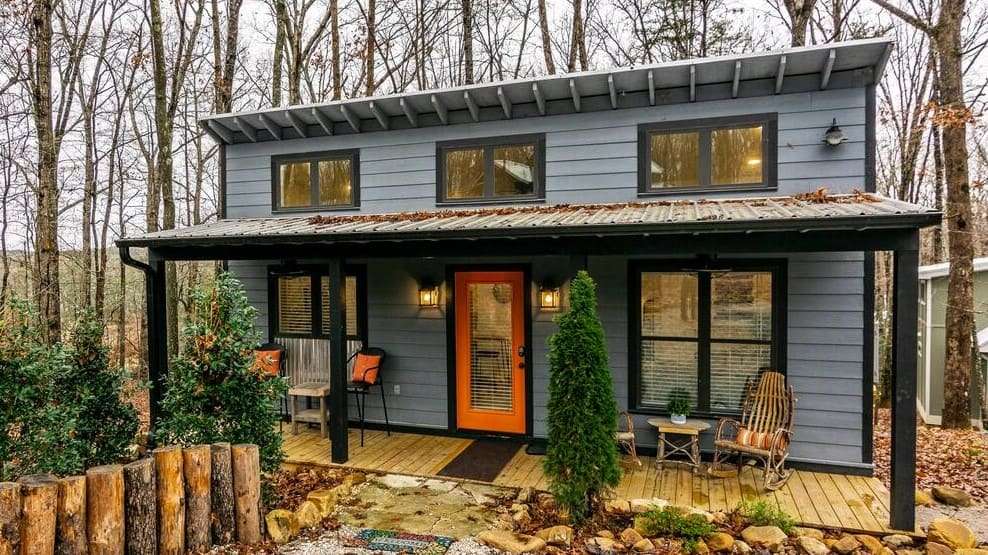This captivating outdoor color photograph, oriented in landscape mode, beautifully captures a two-story rectangular house nestled in the woods. The house is primarily light gray with horizontal Hardy board siding, and features a striking orange front door that has a full glass panel and is outlined with a dark gray frame. Above the door, a silver corrugated tin roof overhangs to form a cozy front porch area without any railing, supported by vertical dark blue posts.

The porch is adorned with a mix of seating options, including a classic wicker rocking chair on the right and a black chair with orange pillows to the left. Brown wood panels line the porch floor, adding warmth to the entrance. Two ornate lanterns flank the door, providing both function and charm. Surrounding the porch is a rocky path, with some rocks visible on the right side and a short span of a rustic wooden fence made of round logs situated on the bottom left of the image.

The house's top level features three short double windows, while the lower level has two sets of double windows, all framed in dark gray. Fallen leaves are scattered across the roof over the porch, adding an autumnal touch. Behind the house, thin, wiry trees stretch upwards, interspersed with glimpses of blue sky, creating a picturesque background that complements the home's serene setting.

Overall, the meticulous details and natural elements blend seamlessly to depict a harmonious and inviting rural residence, captured through the lens of photographic representational realism.